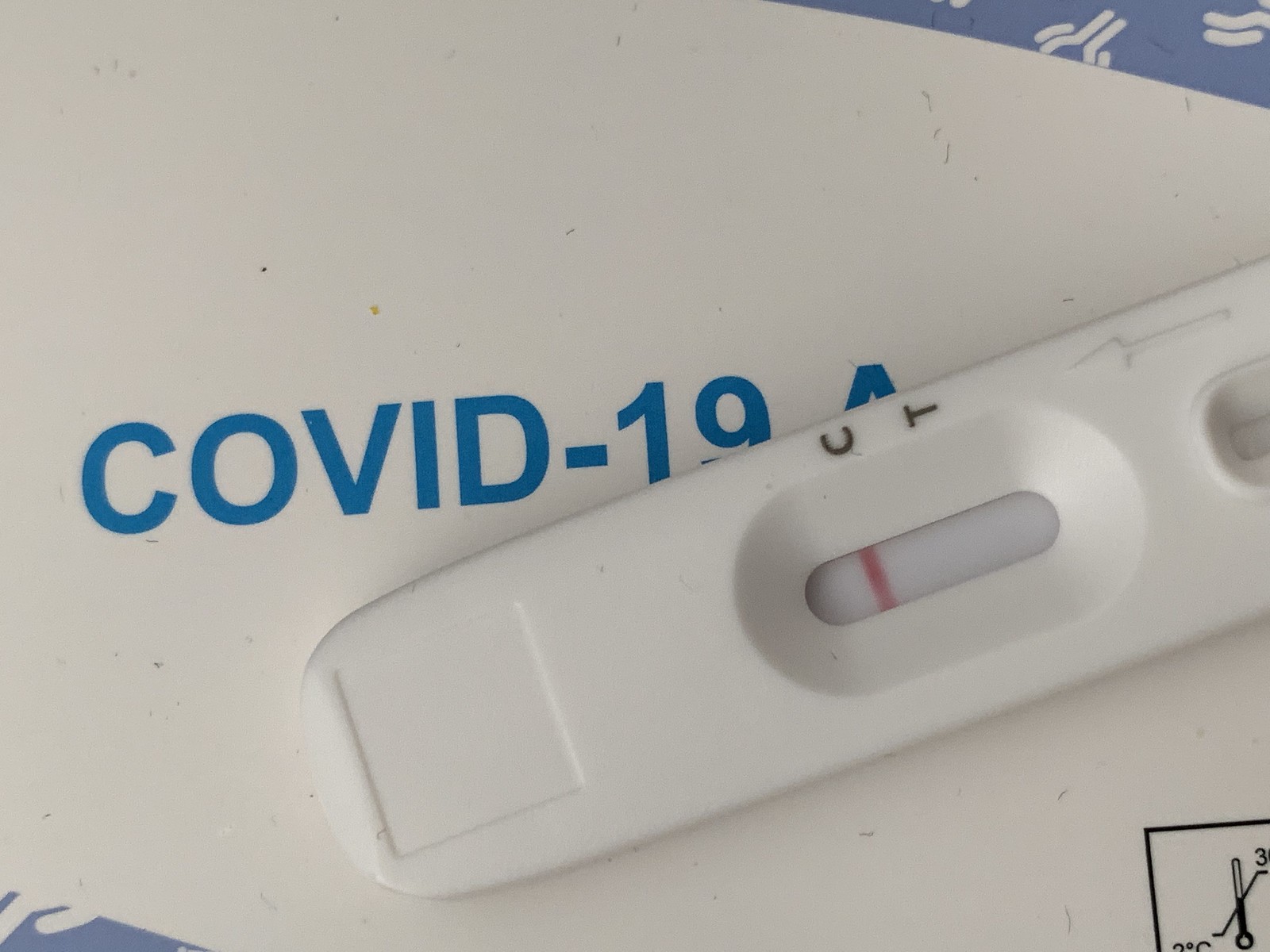The image showcases an early prototype of a COVID-19 test kit. The test kit appears to be made of white plastic, giving it an economical appearance. It is elongated with a rounded end and features an indented square near that end. Prominently displayed on the device are the letters "COVID-19," although part of these letters is obscured by the test unit itself.

A significant feature of the test kit is a red line running through one of the sections next to the labels "C" and "T," which likely indicates the test results. The "C" and "T" markers are accompanied by an upward-pointing arrow. Additionally, there is a small window integrated into the unit.

At the lower part of the test kit, there is a detailed square that appears to include a thermometer icon, displaying a numerical value with a degree symbol, all rendered in stark black and white, resembling pen drawings. This intricate detailing contributes to the overall functionality and design of the test kit, which, despite its seemingly low-cost materials, serves a critical purpose in indicating COVID-19 test results.